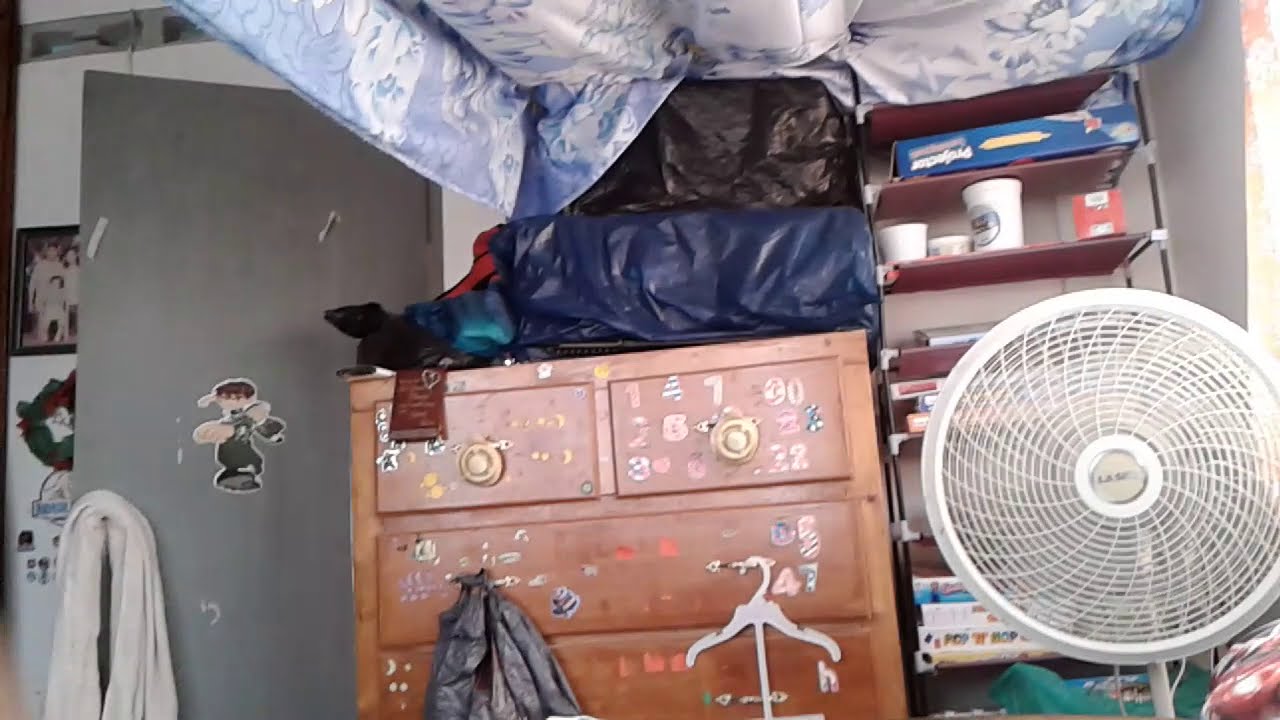This horizontal rectangular photograph depicts a somewhat messy bedroom or storage area, characterized by a central wooden chest of drawers adorned with a multitude of colorful stickers and brass knobs. A hanger dangles from one of the handles of the drawers, which are flanked by large plastic-covered items resting on top. To the right stands a circular-topped white fan with a pole, positioned in front of a cluttered shelf holding coffee mugs, boxes, and other miscellaneous items. On the left side of the image is a slightly ajar gray or brown door, embellished with a cartoon character sticker, and a towel draped over its knob. The white walls in the background feature several picture frames, while a sheet or cloth hangs down from the ceiling, adding to the room's congested appearance.